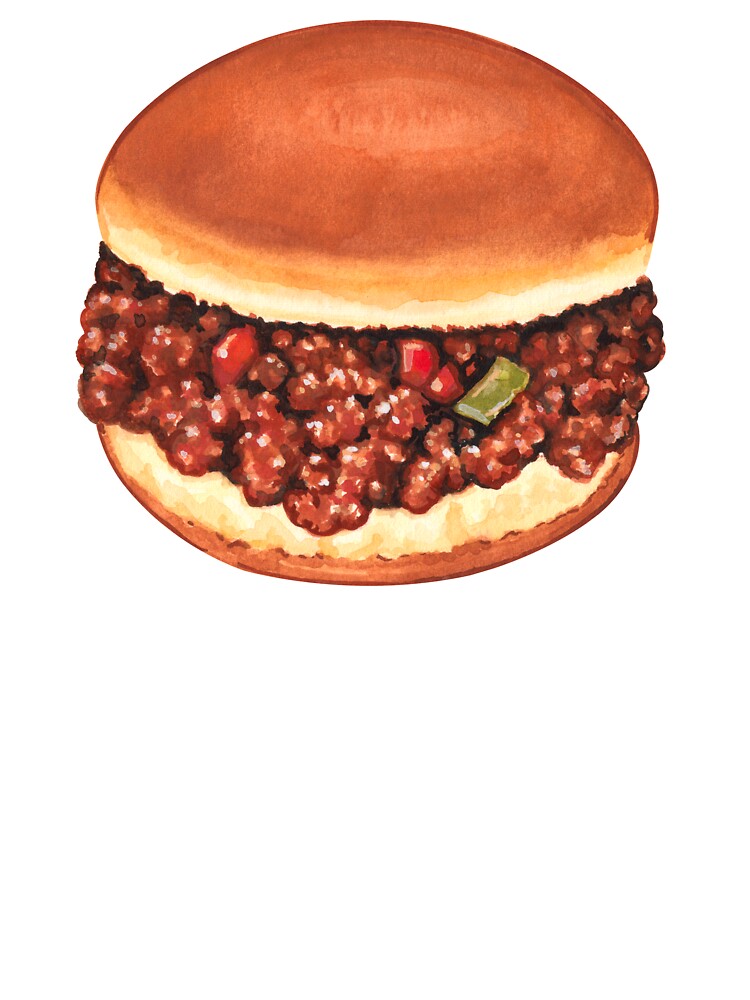This image is an old-style digital rendering of a sloppy joe, featuring a cartoon-like quality. The background is completely white, making the sandwich the sole focus of attention. The illustration showcases a sizable sloppy joe with a brown, fluffy hamburger bun that fades to a lighter color on the inside, indicating a light toasting. The meat mixture inside the sandwich is visibly textured, shiny from the tomato-based sauce, and contains bits of green and red bell peppers alongside small chunks of tomato. The sandwich is depicted head-on, allowing a clear view of both the top and bottom bun, emphasizing the appetizing, slightly shimmery sauce enveloping the crumbled meat. This detailed depiction could serve various purposes—perhaps fitting for a diner menu, a vintage cookbook, or an art piece illustrating classic American comfort food.